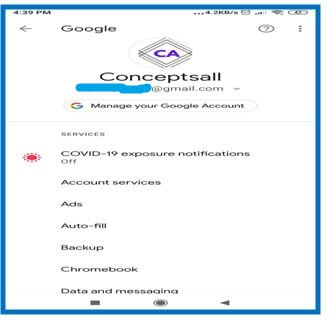The image displays a rectangular digital screen with various elements organized in a structured layout. 

At the top of the screen, "Concept Sol" is written in black text. Above this, there is a multiple-diamond design in purple containing the letters "CA." 

In the top left corner, the word "Google" is visible, with the current time displayed above it as 4:39 PM. The entire display appears elongated and slightly stretched. 

On the top right, the screen indicates a data transfer rate of 4.2 kilobytes per second, alongside icons for an alarm clock, Wi-Fi, and cellular reception. Below these icons are symbols for a question mark and a circle.

Underneath the "Concept Sol" text is an obscured email address ending in "@gmail.com", with the specific address blocked out in blue. Below this, there's a prompt to "Manage your Google account." 

Further down, the screen lists various services. The first item is "COVID-19 exposure notifications," marked as off, accompanied by a red sun icon on the left. Following this in dark grey text are "Account services," "Ads," "Autofill," "Backup," "Chromebook," and "Data and messaging."

The entire page is bordered by a blue rectangular frame, which draws attention to the detailed content within. At the bottom of the screen, additional icons are visible, presumably for navigation or additional options.